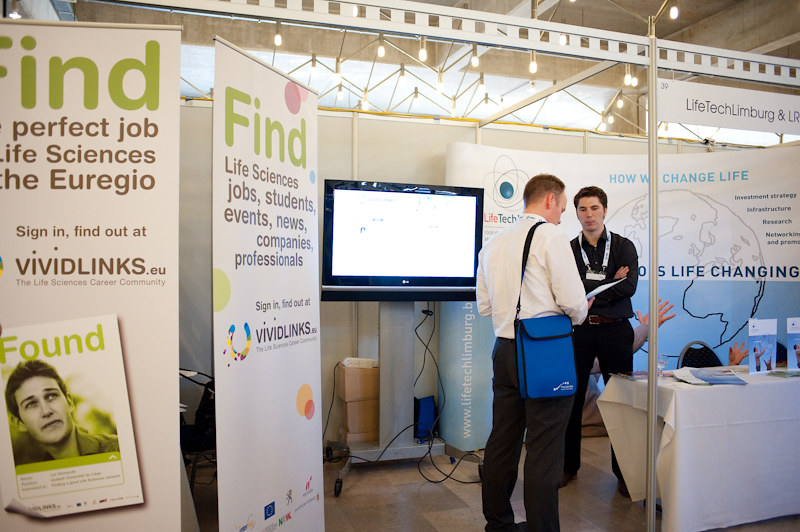This image captures a scene from a science-themed job fair or convention booth. Centrally, two men are engaged in conversation against a backdrop of banners promoting VividLinks, with messages highlighting life sciences, jobs, students, events, news, companies, and professionals. One man, wearing a white collared shirt, black pants, and a blue shoulder bag, stands with his back partially turned to the camera. The other man, dressed in a black shirt, black pants, and a lanyard that suggests he is a representative, faces him. The backdrop includes a black LG television screen on a stand with visible wires and a table covered in a white cloth with pamphlets scattered across it. The environment is lit by white dangling lights and features a tiled floor and scattered cardboard boxes. The scene is set in a glass-enclosed area, hinting at a pop-up shop or exhibit setup.